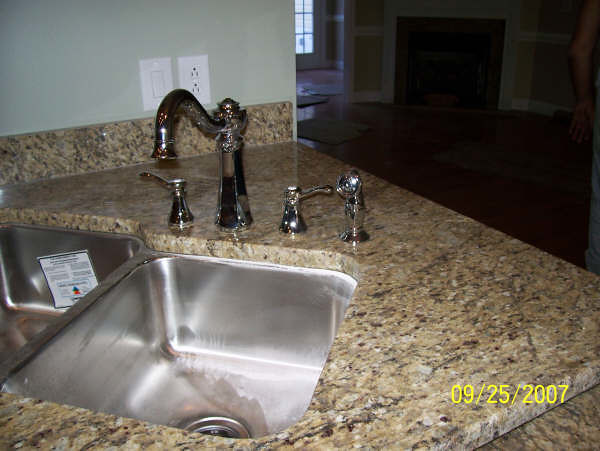The photo features a brand new, angled stainless steel under-counter-mounted sink, distinguished by its high-end design. The sink, which appears to be situated in either a kitchen or bar area of a residence, is equipped with an arching fountain, a spray unit, and separate hot and cold water handles, all of which are of premium quality. The surrounding countertop and splash plate are made of a high-end, stone-like material with a busy, aggregate look reminiscent of granite. Notably, there is still a sticker in the sink, indicating its newness.

In the background, the house appears large and features double doors with multi-pane glass leading to an entryway or foyer area. From the sink, one can view through a hallway into this space, adding a touch of openness to the design. The wall beside the sink showcases a beautiful, higher-end light switch and a double outlet. A timestamp in yellow reading "09-25-2007" is visible in the bottom right corner of the photo.